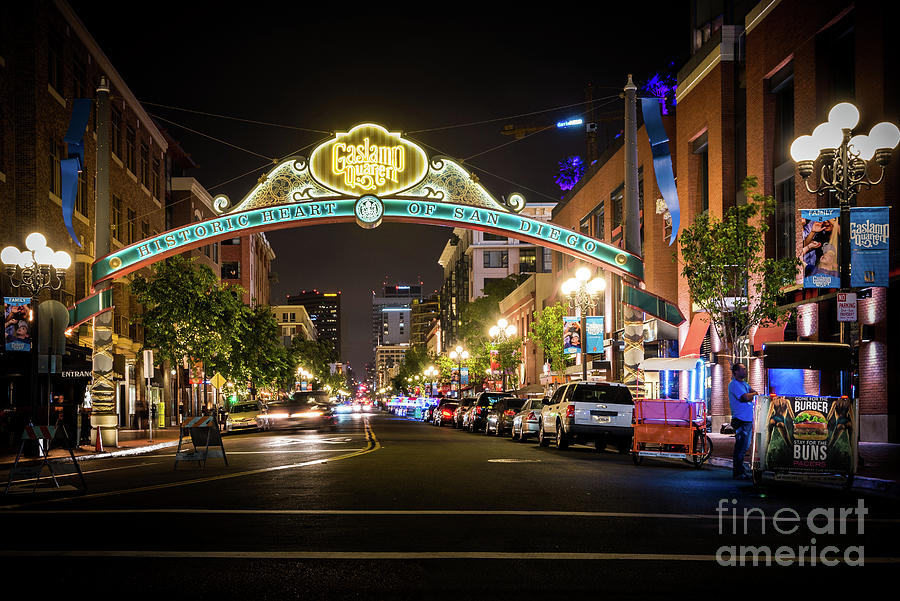In this captivating nighttime photograph of a bustling downtown San Diego street, a large, horizontally aligned, and borderless image showcases the vibrant "Gaslamp Quarter." Dominating the scene is an illuminated arch, stretching from one side of the street to the other. The arch is adorned with two prominent signs: "Historic Heart of San Diego" written in light blue, positioned at the top, and "Gaslamp Quarter" in a classic antique style illuminated with gold neon light beneath it. 

The street is flanked by charming three-story red brick or brownstone buildings, vividly lit up, adding to the picturesque setting. Various businesses, including a hot dog vendor and a "Burgers and Buns" stand, pepper the lively street, elucidating a thriving nighttime economy. Along the road, clusters of streetlights with lit orbs line the sidewalks, and numerous cars are parked along the curbs, emphasizing the popularity of this area.

The top of the photograph reveals a solid black sky, giving a striking contrast to the brightly lit scene below. A grid layout of horizontal and vertical roads frames the city's architecture, with a watermark reading "Fine Art America" subtly placed in the lower right corner of the image. This engaging photograph beautifully encapsulates the essence of San Diego's historic and energetic Gaslamp Quarter.